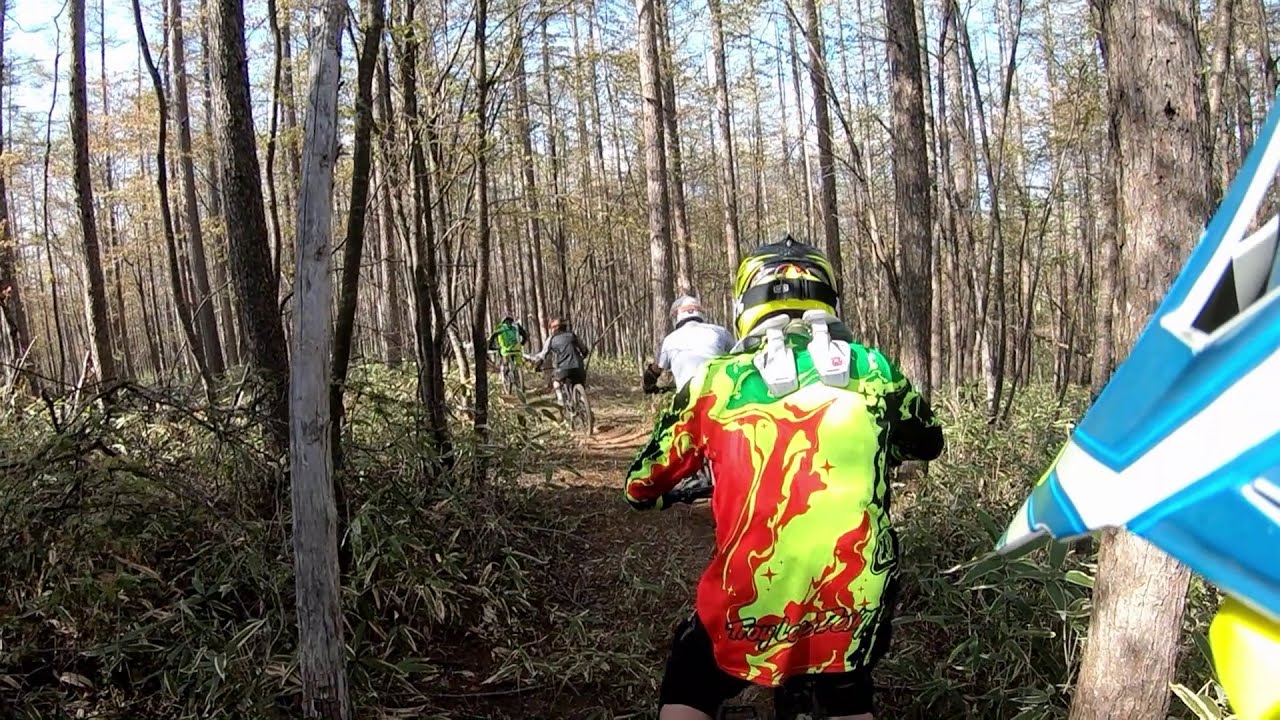This image captures an outdoor setting on a winding dirt bike trail through a densely wooded area, from the perspective of a cyclist. The path, lined with tall trees that have sparse leaves, suggests a late fall or early spring day, as glimpses of a blue sky can be seen through the narrow branches. Traveling down the trail with mountain bikes, the foremost rider in the immediate view wears a striking neon green jersey with splashes of red, complete with long sleeves gripping the bike's handlebars and a black and neon helmet. Ahead, partially visible to the left of this rider, is another cyclist in a white shirt. In the lead, identifiable by a lime green shirt, rides another biker followed by one in a dark-colored shirt. All the cyclists are wearing helmets and are spaced about four to five feet apart. The overall scene suggests a moment of energetic adventure amidst the serene beauty of a forested mountain trail.